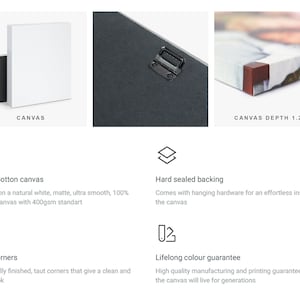A computer screen displays an image with three equally sized pictures across the top. The first picture, labeled "Canvas," features a pristine white canvas. The second picture, slightly larger than the first, shows the back of a black frame with a hook at the top, suggesting it is ready for hanging. The third picture, the same size as the first, focuses on a corner of the canvas with text partially visible, reading "Canvas Depth 1.," with additional details cut off.

Below these images, the screen has a white background divided into four text sections. In the upper left, the text reads, "Cotton Canvas," followed by "Natural White Matte, Ultra Smooth, 100%," and "400 standard," though part of this text is cut off. At the bottom, partially visible text includes, "M-E-R-S," followed by "by finished taunt covers that give a clean," with the remainder obscured. In the upper right, the text states, "Hard Sealed Backing," with a note that it "comes with hanging hardware for an effortless." Lastly, the fourth section, located under the previous text, reads "Lifelong Color Guarantee," promising "high quality manufacturing and printing guarantee" and that the "canvas will live for generations."